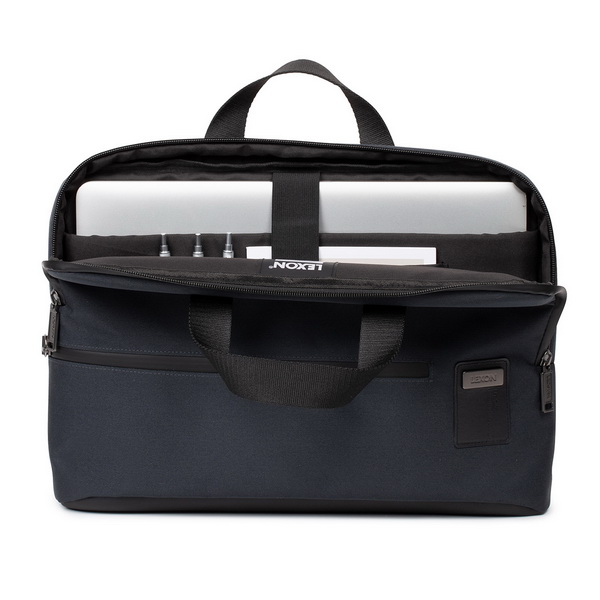The image showcases a navy blue laptop briefcase with black handles and zippers, set against an all-white background. The briefcase is unzipped and open, revealing its contents. Inside, a silver laptop is secured with a black strap in a padded compartment. Below the laptop, there is a pad of white paper. On the left side, the briefcase has slots designed to hold items, currently containing three pen-like objects. A patch on the exterior right side of the briefcase bears the brand name "Lexon" in white letters, and the same branding is prominently displayed inside on a black patch with gray text. One of the black handles is flopped down due to the open briefcase. The overall style of the bag resembles luggage or a professional carrying case.